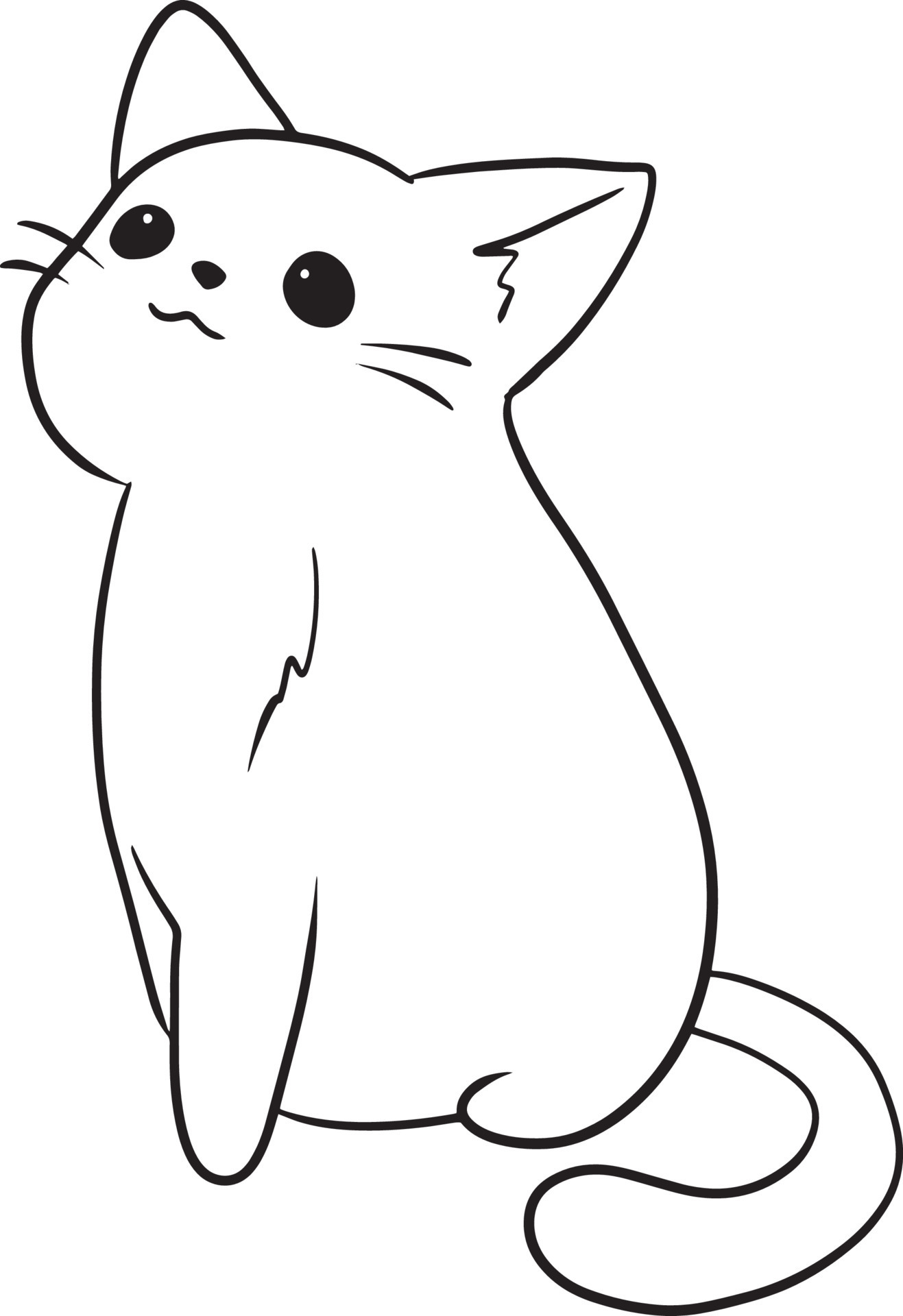This black and white drawing of a cat is outlined in a thin black line on a white background, characterized by simplicity and minimal line work, somewhat akin to images found in a child's coloring book. The cat's body is primarily white, adorned with distinct features in black ink. Its two eyes are black circles with a small white dot at their centers, giving them a focused and expressive look. Below the eyes is a black nose shaped like a curved upside-down triangle, leading down to a thin, mustache-like line representing the cat’s mouth. Four whiskers, two on each cheek, extend outward from the face.

The depiction of the cat’s ears is detailed, with the left ear featuring a line running at a 45-degree angle and a squiggly line underneath to illustrate its inner ear. A similar squiggly line can be found in the middle of the cat’s body, adding to the simplistic charm of the drawing.

The cat’s body posture suggests it is sitting, with its tail curved around towards its back. The left front leg is prominently detailed, while the other legs are less visible, hinting at the cat's sideways orientation. The cat appears to be looking upwards, possibly in anticipation of food or attention. This minimalist, linear drawing has a charming and whimsical quality, capturing a serene and curious feline expression with a few well-placed lines.